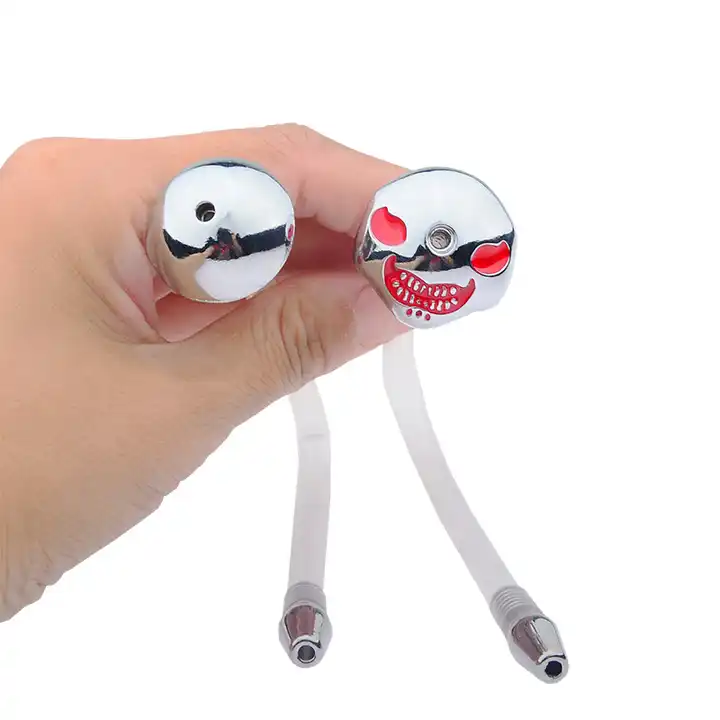The image depicts a fair-skinned hand, likely belonging to a Caucasian individual, emerging from the left side of the frame and holding two objects. These objects have round, silver tops that reflect light, suggesting they are made of stainless steel. Attached to the tops are flexible white hoses, each ending in a metallic nozzle. The overall shape and design of the objects make their specific purpose unclear, potentially resembling nozzles, pens, or adult toys. The nozzle on the right features a sinister, carved face with two red eyes and a wide, menacing grin. The image background is entirely white, providing no additional context or identifying marks to determine the exact nature or function of the objects.